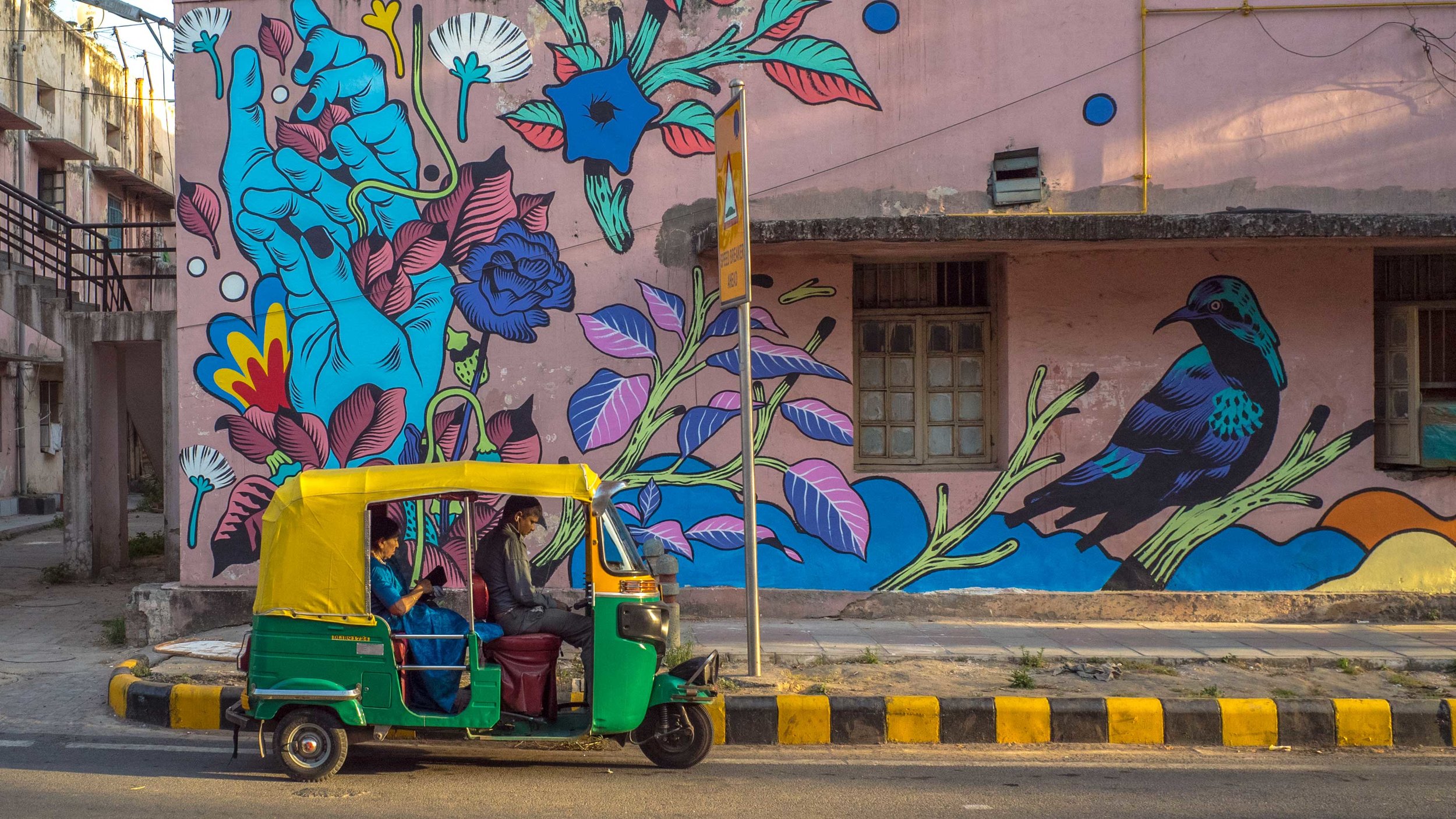This photograph captures a vibrant street scene in a small, non-American town. The image appears to be taken from a sidewalk looking across the street. A distinctive green three-wheeled tuk-tuk with a yellow tarp top is parked along the curb. The tuk-tuk has a man in the driver's seat, dressed in a tuxedo and hat, and a woman in the back, wearing a blue dress. The sidewalk is made of concrete and features a curb painted in alternating black and yellow stripes.

Dominating the background is a pinkish building adorned with a striking and colorful mural. The mural is rich in floral motifs, depicting blue hands surrounded by purple and blue leaves and petals. There are also flowers with green and red leaves. On the right side of the mural, a bird, which might be a crow, colored in shades of blue and turquoise, is perched on a branch. The artwork has an abstract feel, adding a vibrant and artistic flair to the scene.